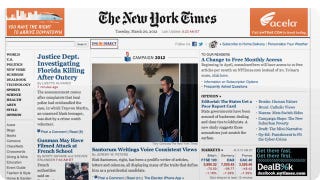This screenshot captures the digital edition of the New York Times. The page features a prominent orange advertisement on the left side, although the text within the ad is blurry and unreadable. A similar orange ad from Asilar is positioned on the right side, but its text remains unclear even when zoomed in. Prominently displayed on the left side is a headline: "Justice Department Investigating Florida Killing After Outcry," accompanied by a photo of three people standing in front of a wall, although the title of this specific article is too blurry to decipher.

In the top right corner, there is a section labeled "I change," related to some airline information, though specific details are unreadable. Additionally, the right side includes a column section and a markets box, and at the bottom right corner, there is a DealBook ad on a black background. Directly beneath the New York Times banner, there are visible icons for Facebook and Twitter, indicating options for social media sharing. Despite the detailed layout, much of the text throughout the page remains indistinct and challenging to read.